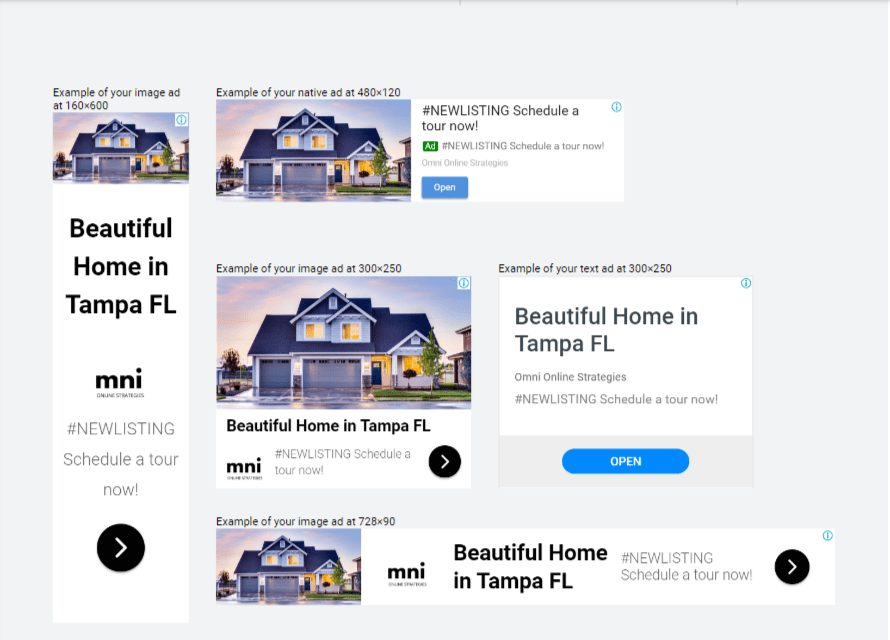This is a detailed screenshot showcasing examples of ads that will be displayed on a website, all set against a grey background. 

1. **First Ad (Left Side):** 
   - **Type:** Image Ad
   - **Dimensions:** 160 by 600 pixels (vertical, slim section)
   - **Content:** 
     - **Top Section:** Features a photo of a two-story home. The upper floor has two windows, while the ground floor includes two garage doors, a main door, and a main window.
     - **Text:** "Beautiful moment in Florida, MNI, #newlistings" which functions as a button.

2. **Second Ad (Right Side, Top):** 
   - **Type:** Native Ad
   - **Dimensions:** 480 by 120 pixels
   - **Content:** 
     - **Image Location:** Left side.
     - **Text (Right Side):** "#newlistings, schedule a tour now" in white text on a green background. Below it includes "Omex Online Strategies" and a blue button labeled "Open."

3. **Third Ad (Below Second Ad):** 
   - **Type:** Image Ad
   - **Dimensions:** 300 by 250 pixels
   - **Content:** 
     - **Top Section:** Main photo.
     - **Text (Bottom):** "Beautiful moment in Florida, MNI, #newlistings, schedule a tour now," accompanied by a black button.

4. **Fourth Ad (Right Side, Below Third Ad):** 
   - **Type:** Text Ad
   - **Dimensions:** 300 by 250 pixels
   - **Content:** 
     - **Text Only:** "Beautiful moment in Florida, Omex Online Strategies, #newlistings, schedule a tour now," with a blue button at the bottom.

5. **Fifth Ad (Bottom of the Screenshot):** 
   - **Type:** Image Ad
   - **Dimensions:** 728 by 90 pixels
   - **Content:** 
     - **Image Location:** Left side.
     - **Text:** "Beautiful home in Tampa, Florida" highlighted in bold black text, followed by "MNI" and "#newlistings, schedule a tour now," with a black button on the right.

Each ad is carefully designed to promote real estate listings, featuring a mix of images and compelling calls to action, ensuring users are encouraged to engage and explore the listings further.